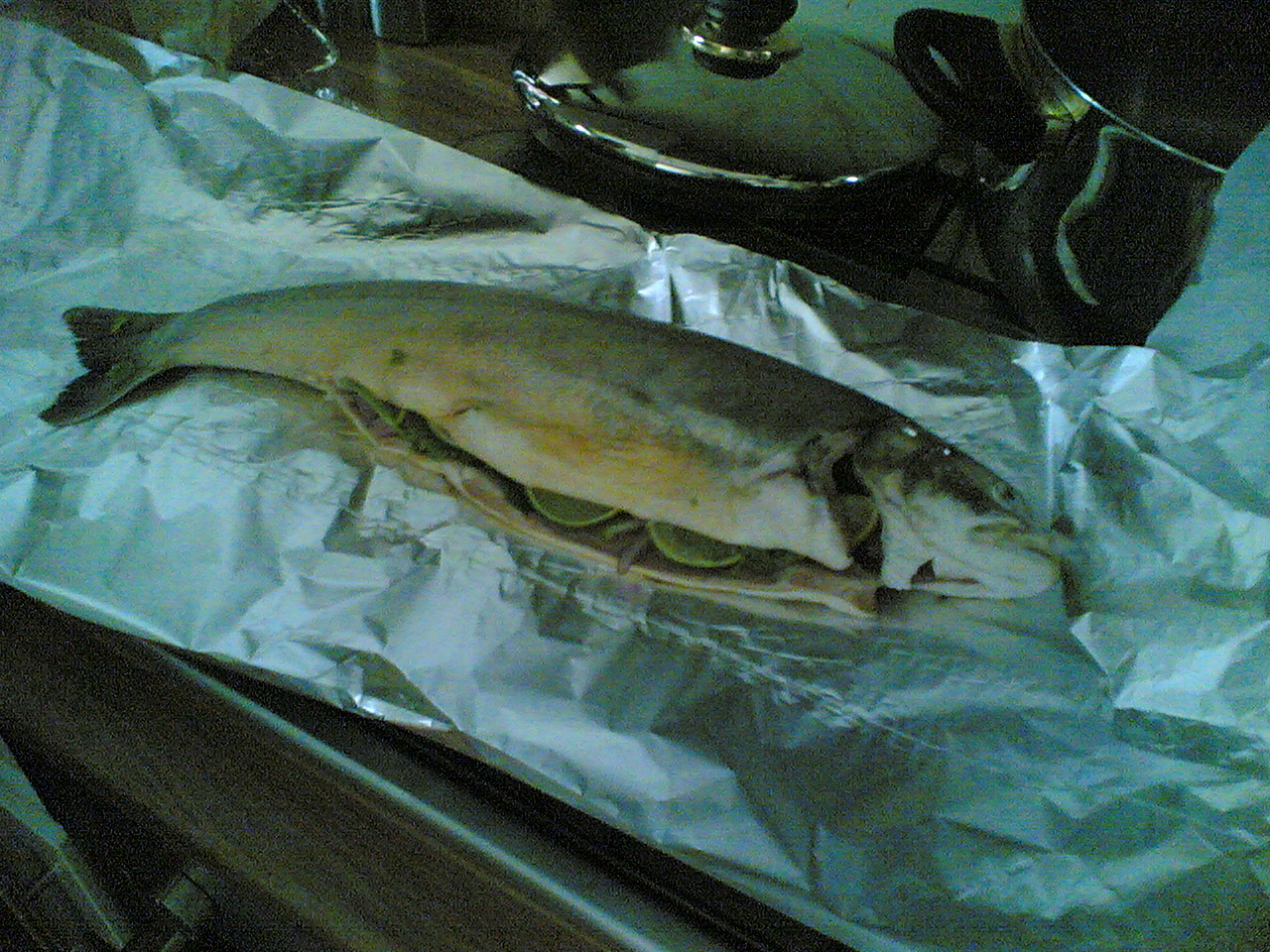This image captures a low-resolution, pixelated photograph of a medium-sized, light gray-silver fish being prepared for cooking. The whole fish, with its head and tail intact, lies gutted and stuffed with lime, onions, various herbs, and possibly other citrus items on a large sheet of aluminum foil, suggesting it will be wrapped and cooked. The scene is set in a kitchen, as evidenced by the stainless steel pot and lids visible in the background. The fish rests on a countertop, which may be made of wood, with the edge of what appears to be an oven dial and door glimpsed in the lower left of the image. Despite the pixelation and image artifacts, the focus clearly remains on the culinary preparation of the fish.